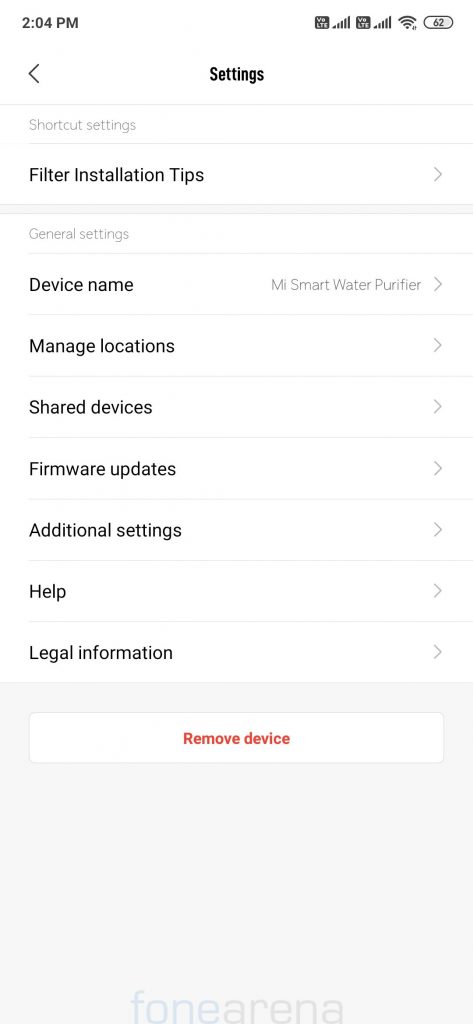The image portrays a smartphone screen displaying an app page for the Mi Smart Water Purifier settings. At the top of the screen, there is a status bar showing the time (2:04 PM) on the top left, and icons for battery, WiFi, and dual SIM (VoLTE) on the top right. Below the status bar, the page title "Settings" is prominently displayed in black text.

Beneath the title, the page is sectioned into various categories. The first section, "Shortcut Settings", features installation tips for quick access. Following this, the "General Settings" section includes the device name, listed as "Mi Smart Water Purifier". Further options available in this section are "Manage Location", "Shared Devices", "Firmware Updates", "Additional Settings", "Help", and "Legal Information".

At the bottom of the page, there is a button labeled "Remove Device" in brown text, set against a white background. Below this button, in the footer, the text "FONE arena" is displayed, with "FONE" in light blue and "arena" in dark grey. The footer background is grey, while the backdrop for the entire page is white. Additionally, a back button is situated on the top left of the screen, next to the "Settings" title, offering navigation to the previous page.